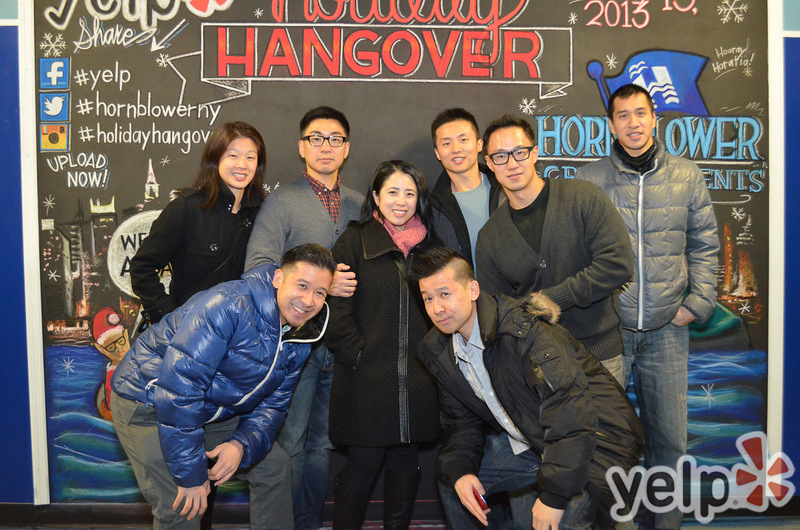The photograph is a detailed color image taken in landscape orientation, featuring a group of eight Asian individuals posing together. The subjects are dressed appropriately for the winter season, mostly in coats, indicating the colder weather. They consist of a row of people standing shoulder-to-shoulder at the back, with two individuals crouching and smiling in the front, creating a sense of camaraderie. Most prominent among them is a young woman at the center, clad in a black overcoat, her brown hair framing her smiling face. 

To her left, a man in a blue puffer jacket and gray pants stands next to a woman with brown hair, also smiling warmly. Beside her is a man with glasses, black hair, and a layered outfit featuring a gray sweater over a red plaid shirt. 

The group is positioned in front of a large, detailed chalkboard-like sign filled with holiday-themed illustrations including a skyline over water and a festive figurine in the water wearing a holiday hat. Dominating the backdrop is the phrase "HOLIDAY HANGOVER," written in striking red letters with a white drop shadow. Numerous social media icons and hashtags accompany the text, alongside logos for Yelp and Hornblower Cruises New York. The Yelp emblem is notably present in both the upper left corner and the bottom right corner of the backdrop. The overall style of the image is photographic representational realism, capturing both the joyful expressions of the subjects and the intricate design of the festive backdrop in clear, precise detail.